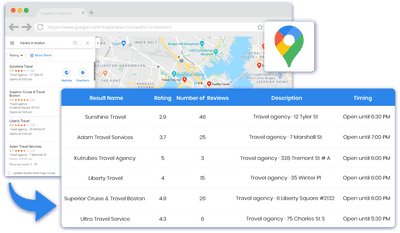The image displays the top results of a Google search for travel agencies. The results appear within a gray and white box. At the very top, there is a blue section containing white text indicating the search category and related results. The listings provide detailed information about various travel agencies, including their names, ratings, number of reviews, descriptions, and opening hours.

1. **Sunshine Travel**: This agency has a rating of 2.9 based on 46 reviews. It is a travel agency and is open until 6:30 PM.
   
2. **Atom Travel Services**: Rated 3.7 with 25 reviews, this travel agency operates until 7:00 PM.
   
3. **Qutrubis Travel Agency**: With an impressive rating of 5.0 from 3 reviews, this agency is open until 6:00 PM.
   
4. **Liberty Travel**: This travel agency boasts a 4-star rating from 15 reviews and is open until 6:00 PM.
   
5. **Superior Cruise and Travel**: Holding a high rating of 4.9 based on 26 reviews, this agency is open until 6:00 PM.
   
6. **Ultra Travel Services**: This agency has a 4.3 rating with 6 reviews and closes at 5:30 PM.

The detailed information provided for each travel agency includes their operational hours, making it easier for users to choose the best option based on ratings and reviews.